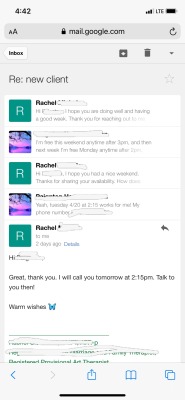The image is a detailed screenshot from Google Mail, labeled as "mail.google.com" at the top. It captures an email conversation between Rachel and an unnamed recipient, with parts of the conversation, such as the date, time, and the recipient's name, obscured. The communication shows Rachel replying three times and the recipient responding twice. 

Rachel's icon features a white "R" on a green background, while the recipient's icon is a purple image, though its details are indistinguishable. Towards the bottom of the screenshot, Rachel's message is open and readable; it states, "Great, thank you. I will call you at 2:15 PM. Talk to you then. Warm wishes," followed by a blue butterfly emoji. The interface also displays a back arrow in the bottom left-hand corner and an options button in the bottom right-hand corner.